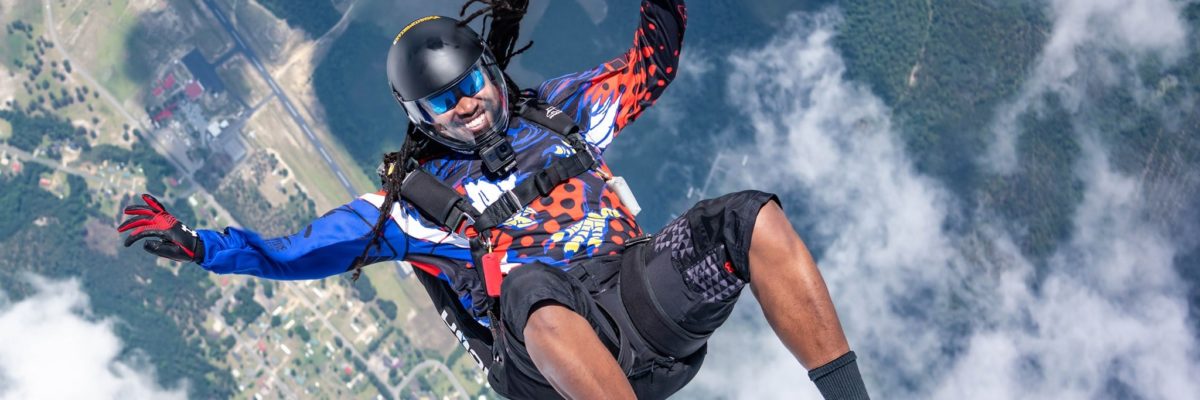The vibrant color photograph captures a breath-taking skydiving moment, viewed from above in a landscape orientation. The smiling man, clad in a black helmet and blue sunglasses, is falling with his back toward the earth and his limbs spread wide. His long-sleeved blue jacket, adorned with striking orange and white patterns, and black knee-length pants contrast against the green patchwork landscape below. He is also wearing black socks and gloves, with skydiving equipment strapped securely to his chest and legs. White clouds float on the right side of the image, underneath which stretches a blend of green fields, wooded areas, and buildings, offering a magnificent earthward view. The photo, likely taken by a fellow skydiver or a GoPro, captures this exhilarating descent in vivid detail.